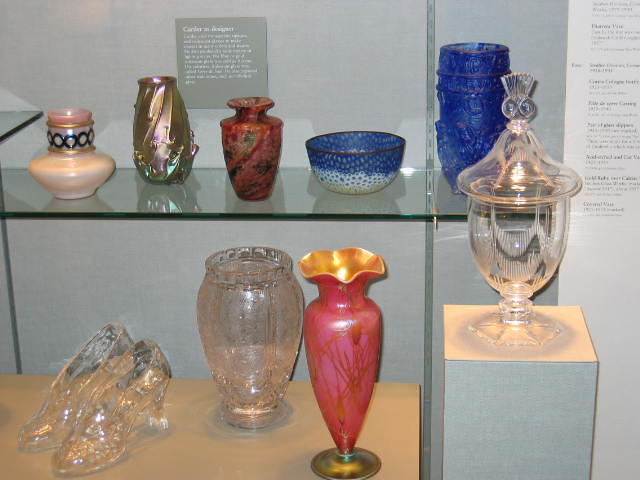This photograph captures a detailed display in a museum showcasing an array of vases and glass items. The eclectic collection is arranged on two glass shelves and a white pedestal. The backdrop is a gray wall adorned with a plaque featuring white text, presumably describing the artifacts, though the writing is too small to discern. 

On the top shelf, from left to right, there's a cream-colored vase with blue circles around its neck, followed by a taller, iridescent vase. Next is a short, reddish-brown vase with a narrow opening. Adjacent to these is a blue bowl with a white base and blue dots. Completing the top shelf is a large dark blue vase. 

The bottom shelf showcases a unique pair of glass slippers, reminiscent of Cinderella's, alongside a large pinkish-glass vase. Further to the right sits a red vase with a gold interior, which has a wavy, textured exterior. On a white pedestal below, there is an ornate lidded glass vase or candy holder. 

In front of the shelves on a white table are two additional vases: one clear with gold accents and another red-pink glazed with gold. The elaborate display includes clear plastic and glass items, with notable pieces such as a peach vase, metallic brown vase, and a cobalt-blue vase rounding out the collection.